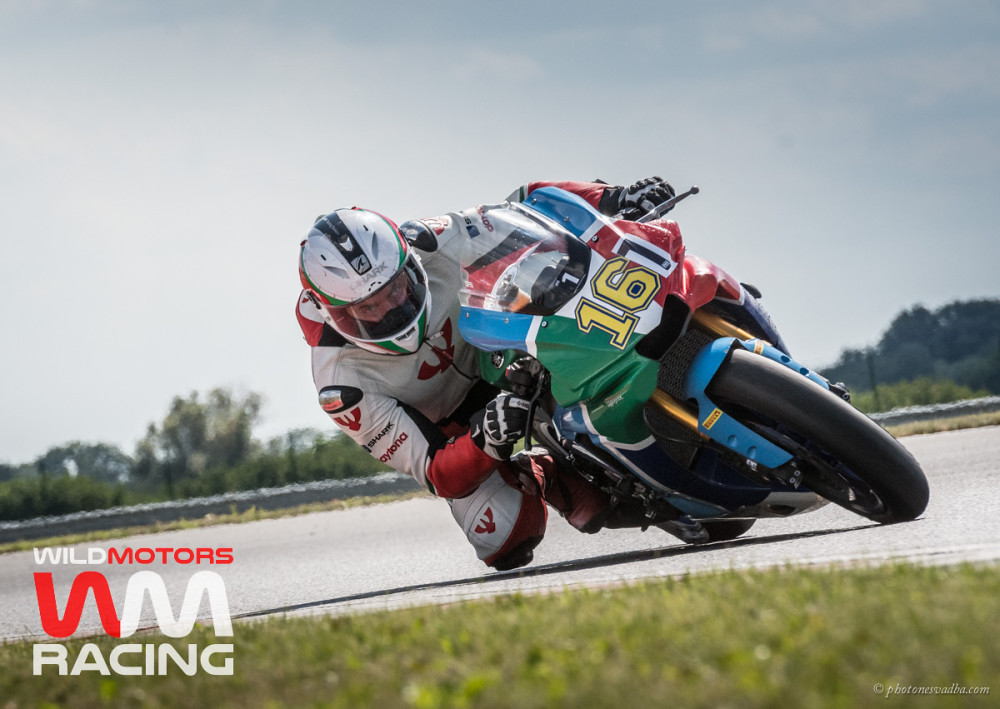The image captures a dynamic outdoor scene of a motorcycle racer mid-turn on an asphalt racetrack bordered by grass, trees, shrubbery, and a guardrail in the distance under a cloudy sky. The racer, clad in a white racing outfit adorned with various sponsor names, and equipped with gloves and a white helmet featuring a blue or black central stripe, is leaning his bike sharply to the right, with his knee nearly touching the ground. His motorcycle is multicolored with blue, red, green, and white segments and bears the number 161, where the '1' within the '6' is gold, and the second '1' is black. Strikingly, the image includes the "Wild Motors" branding in the lower left corner, showcasing a seamless red and white interconnected 'WM' logo, followed by the word 'Racing'. The bike is equipped with a windshield, and the racer appears to be in a fast-paced race environment, highlighting the intensity and skill of the sport.